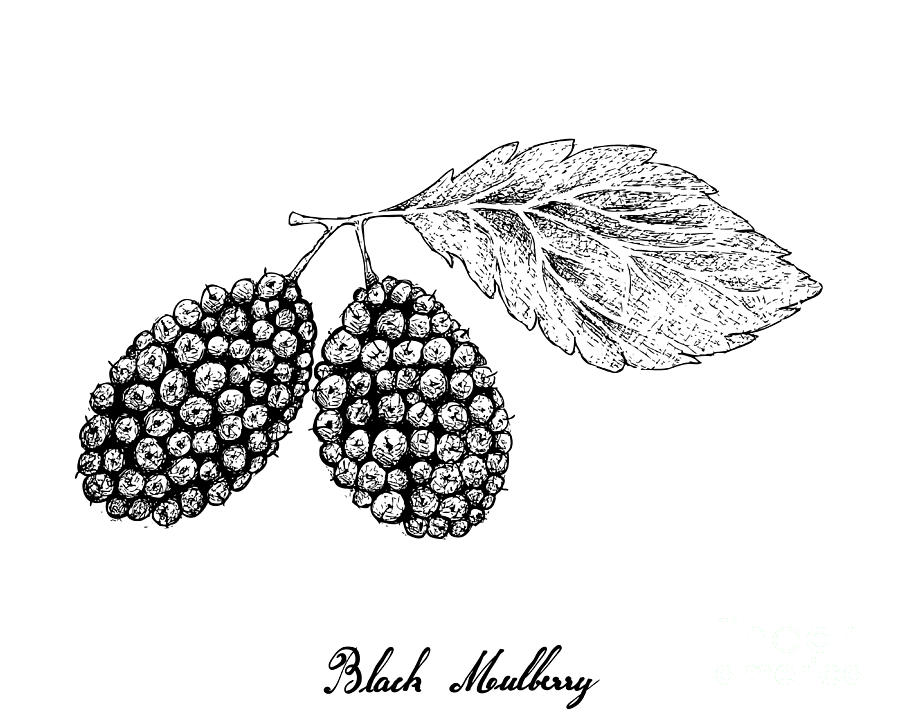This black-and-white illustration, reminiscent of scientific textbook artwork, depicts a detailed rendering of the black mulberry. Set against a white background, the drawing showcases two oval-shaped mulberries hanging from a short stem, accompanied by a single serrated leaf. The intricacy of the leaf's veins is meticulously captured, giving it depth and texture. Each mulberry consists of numerous tiny, spherical nodules clustered together, similar to raspberries but forming a larger oval shape. The use of shadow work highlights the individual berries, enhancing the textural realism of the fruit. Below the illustration, "black mulberry" is elegantly inscribed in black script font, adding a refined touch to the botanical depiction.